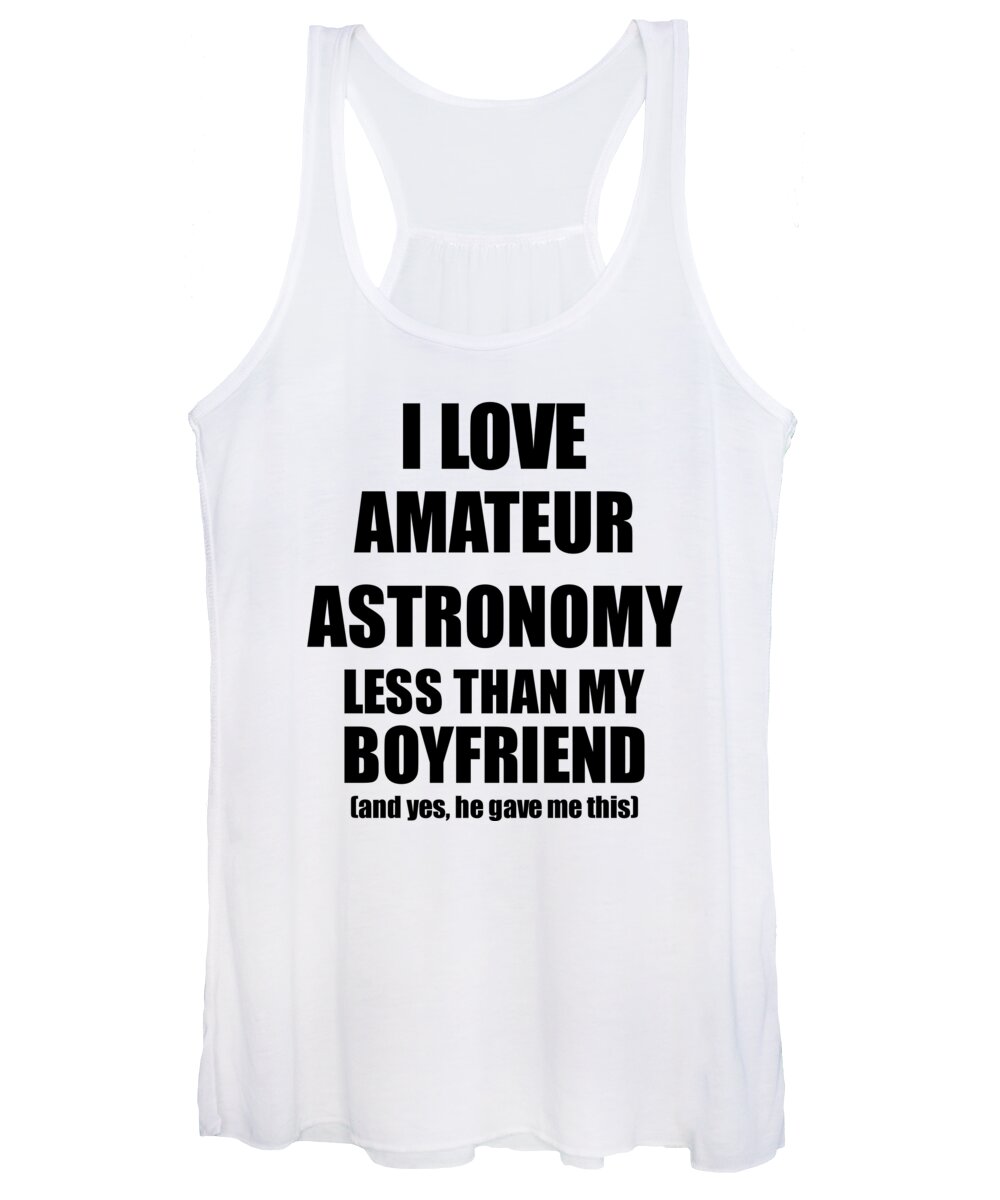This product photograph, ideal for a commercial listing or catalog, showcases a pristine, white, thin-strapped cotton tank top against a completely white background. The tank top features bold black text prominently displayed on its front. The message, spread across multiple lines, reads: "I love amateur astronomy less than my boyfriend." This is followed by a smaller, playful comment in parentheses at the bottom: "(And yes, he gave me this)." The tank top appears new, with a bright white hue and natural folds that give it a slightly wrinkled, dynamic look as it hangs, enhancing its presentation.